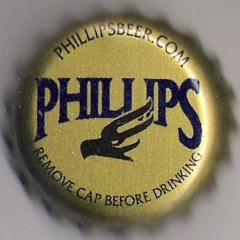The photograph depicts a close-up view of a gold beer cap prominently labeled with "PhilipsBeer.com" repeatedly around its perimeter in small letters. The central text "Philips" is showcased in large, navy blue letters that slightly curve upwards and downwards, and is accompanied by a black emblem resembling a flying bird, possibly an eagle or a bird in flight. Below this, a clear message advises "remove cap before drinking." The cap, recognizable by its jagged, wavy edges typical of pry-off bottle caps, is set against a neutral gray background. The overall image appears somewhat blurred but focuses solely on the cap itself, emphasizing its details without providing context such as location, time, or the rest of the bottle. The photograph is relatively small, measuring approximately one and a half by one and a half inches.